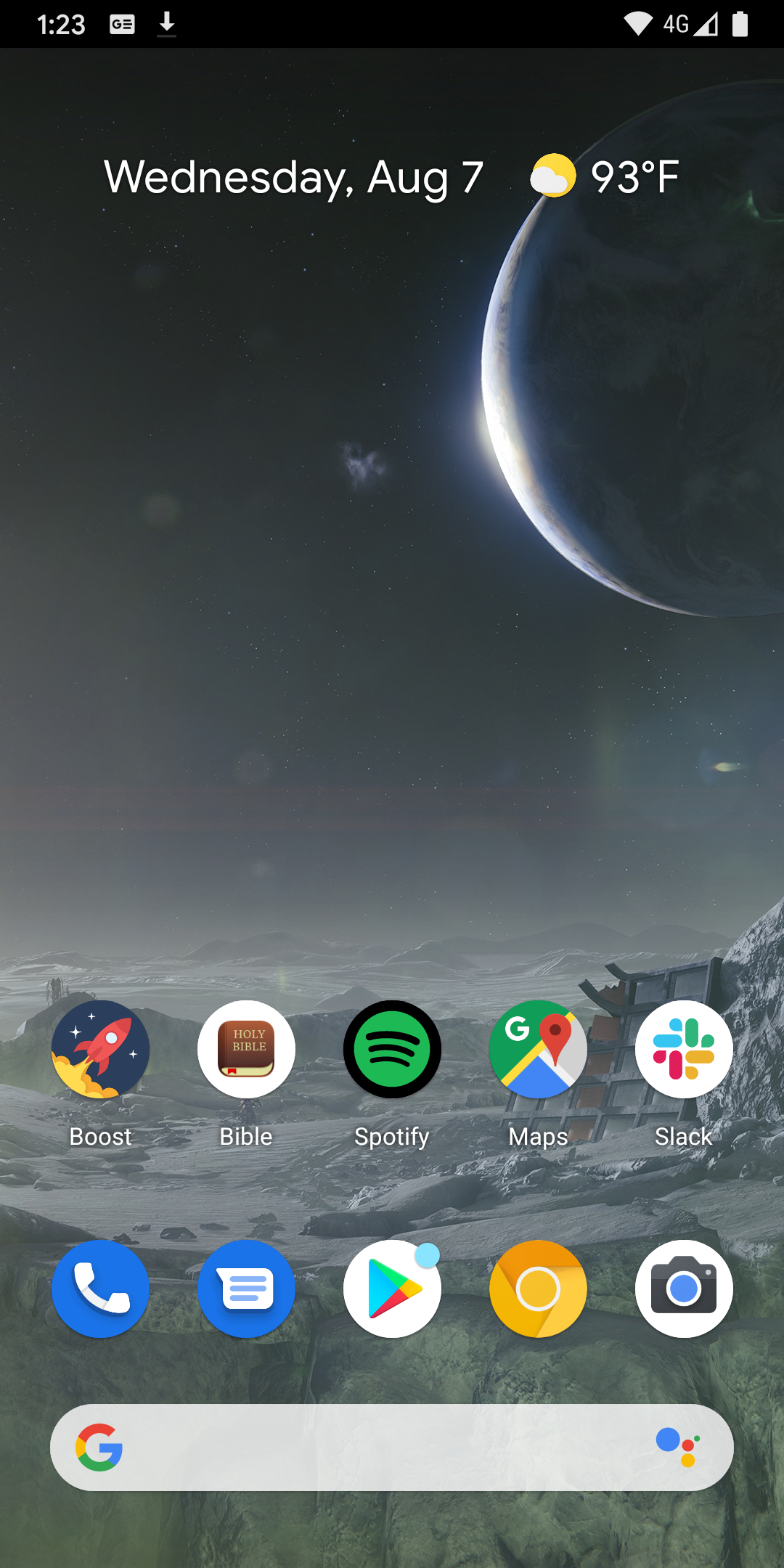This is a detailed caption of a smartphone screenshot showcasing the home screen. The time displayed at the top left is 1:23, and the battery icon at the top right is almost full, with no indication of depletion. The current date is shown as Wednesday, August 7th, accompanied by the weather information which reports partly cloudy conditions with a temperature of 93 degrees.

The phone's wallpaper is a striking image depicting a lunar or planetary surface at the bottom, characterized by its gray, rocky texture. The upper portion of the background transitions into the vast expanse of outer space, punctuated by a celestial body resembling a planet. This planet is partially illuminated by the sun on its left side, casting the rest into shadow, lending the scene a moody, cosmic ambiance.

The screen layout features two rows of app icons at the bottom. The first row includes, from left to right: Boost, Bible, Spotify, Maps, and Slack. The second row, situated directly beneath, contains: Phone, Messaging, App Store, Google Chrome, and Camera. These apps are neatly arranged, reflecting the user's preferences and daily utilities.